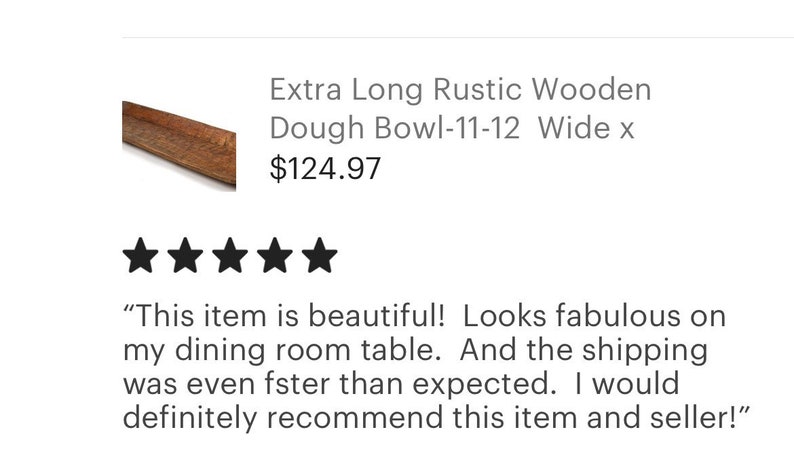Screenshot Description: Extra Long Rustic Wooden Dough Bowl

The screenshot displays an item for sale with a white background and no distinct borders, except for a thin, very light gray line at the top edge. In the upper left-hand corner, there is a small inset photograph of what appears to be a piece of wood, indicating the item is a wooden dough bowl, though it looks relatively flat.

Next to the image, in gray typeset, the text reads: "Extra Long Rustic Wooden Dough Bowl, 11-12 Wide X." Below this, the price is listed in bold black type as $124.97. 

Underneath the price, five stars are arranged in a vertical line, all filled in black, indicating a five-star rating. 

Following the rating, in a slightly darker text than the heading, a user review reads: "This item is beautiful. Looks fabulous on my dining room table. And the shipping was even faster than expected. I would definitely recommend this item and seller."

This screenshot indicates that the Extra Long Rustic Wooden Dough Bowl is highly rated and comes with a positive customer review, praising both the item itself and the prompt shipping service.